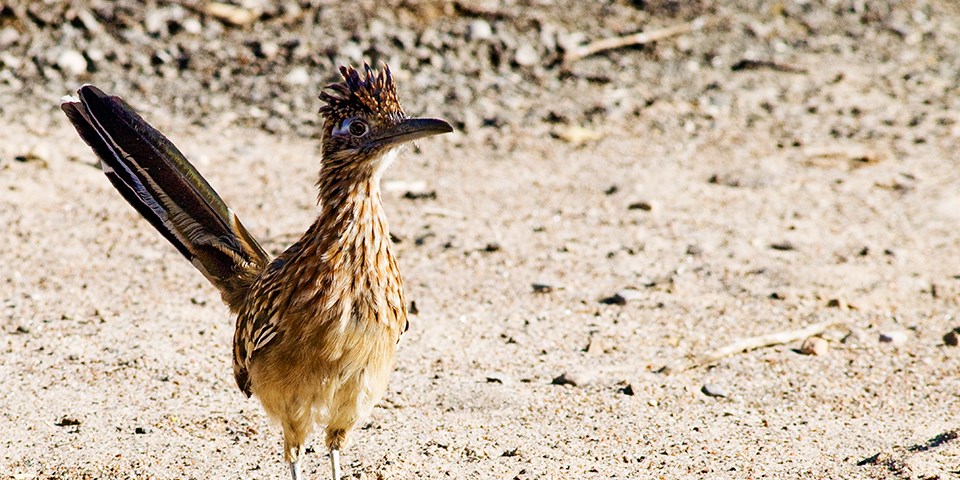This close-up photograph captures a roadrunner standing in a sandy, featureless terrain. The bird occupies the left half of the frame, its gaze directed slightly to the right of the camera with an alert and curious expression. The roadrunner's prominent brown crest resembles spiked hair or a mohawk, complementing its long, dark-colored beak. One of its eyes makes direct eye contact with the viewer, enhancing the photograph's intensity. The lower part of its body displays lighter feather tones transitioning to bare white legs, which are not fully visible in the image. Noteworthy is its large, stiff tail, almost the length of its body, fanning out towards the left side. The bird's coloration is a mix of brownish hues with speckles of black, creating a rich, mottled texture. The sandy ground is pale yellow, consistent with the exposure brightness, and the out-of-focus darker rocks in the background add depth to the scene.